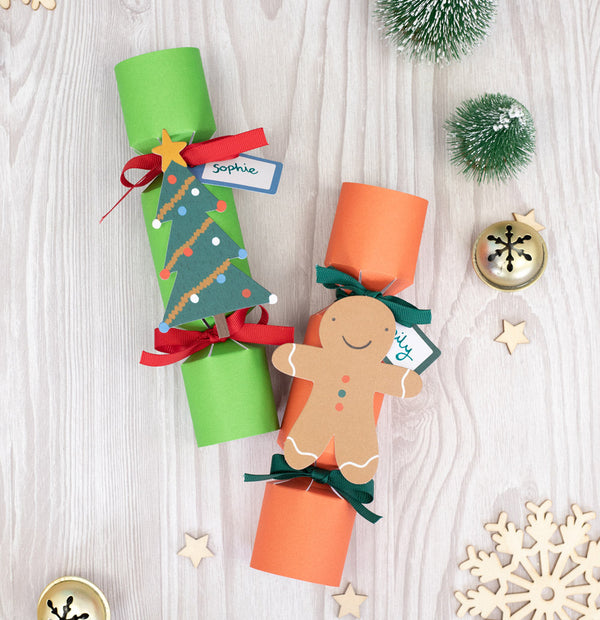The image depicts a detailed, festive holiday scene on a whitewashed wood plank table. At the center are two Christmas crackers. The first cracker, wrapped in orange paper with dark green ribbons, is adorned with a gingerbread man cutout and a nametag inscribed with "Emily." The second cracker, in green paper with red ribbons, features a Christmas tree cutout and a nametag that reads "Sophie." Scattered around the table are various holiday-themed decorations: two golden brass jingle bells, one positioned in the upper right and the other in the lower left, a cutout snowflake in the lower right, along with four stars, and a few miniature bristle pine trees dusted with artificial snow, reminiscent of those seen in model railroad exhibits. The overall arrangement is viewed from above, providing a clear, festive tableau.